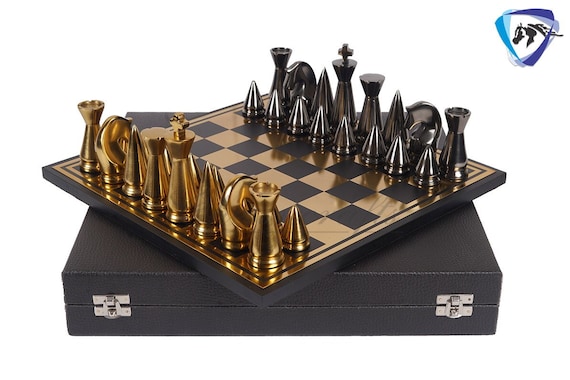The detailed image depicts an exquisitely designed animation featuring a luxury chessboard displayed on top of a sleek black briefcase. The chessboard, which is angled diagonally in the shape of a diamond, alternates between shimmering gold and glossy black (obsidian-like) squares. The chess pieces are similarly divided, with gold pieces arranged on the bottom left and dark metallic (obsidian) pieces on the top right. The board's border and thickness are also black, adding to the premium feel of the set. The foreground reveals two silver hinges of the briefcase, indicating its secure construction. The background is a solid white, emphasizing the chessboard. In the top right corner of the image, a logo featuring an upside-down triangle in hues of light blue, blue, purple, and light purple is present, adding a touch of brand identity. This refined, visually striking setup suggests the product is likely high-end and exquisitely crafted.